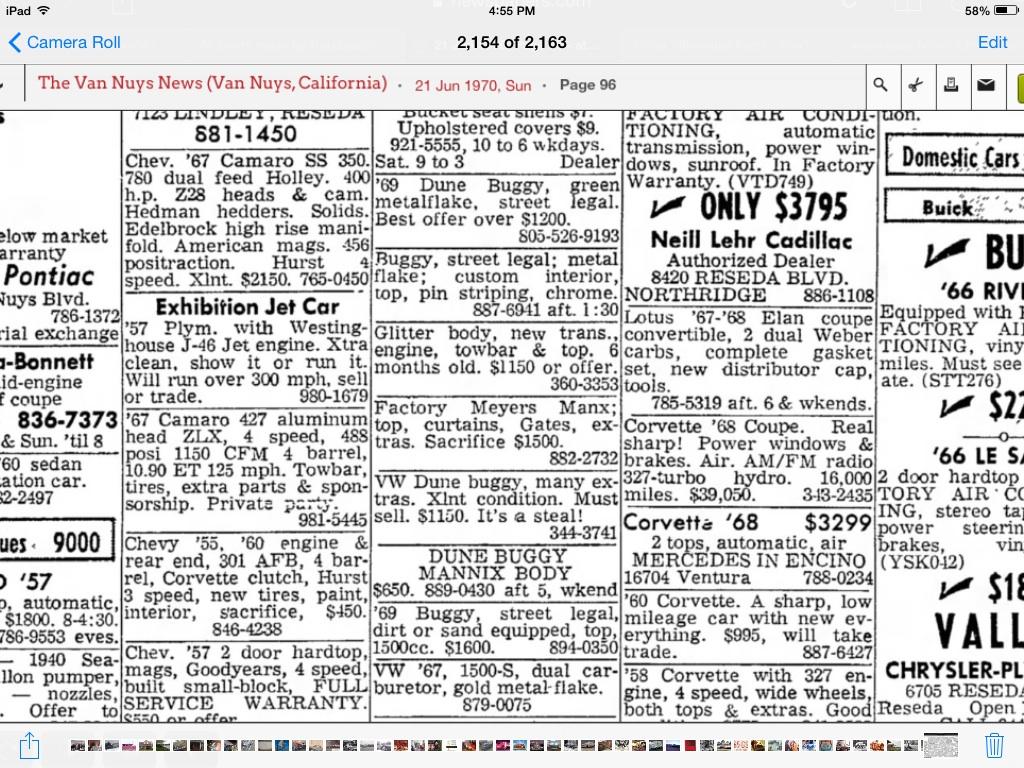This detailed black and white newspaper advertisement is a screenshot from the camera roll of an iPhone, captured at 4:55 p.m. The primary image is an original 1970s "For Sale" section from the Van Nuys News in Van Nuys, California, dated June 21, 1970, on a Sunday. The prominently displayed page, possibly page 96, lists various cars for sale, including models like a 1968 Corvette and a 1967 Camaro. Each vehicle is meticulously organized within individual square sections, providing details such as the make, model, phone number, and price. The screenshot also includes the iPhone's interface at the bottom, showing thumbnails of other images in the camera roll, along with options to share or delete the image, marked by a trash can icon on the bottom right.